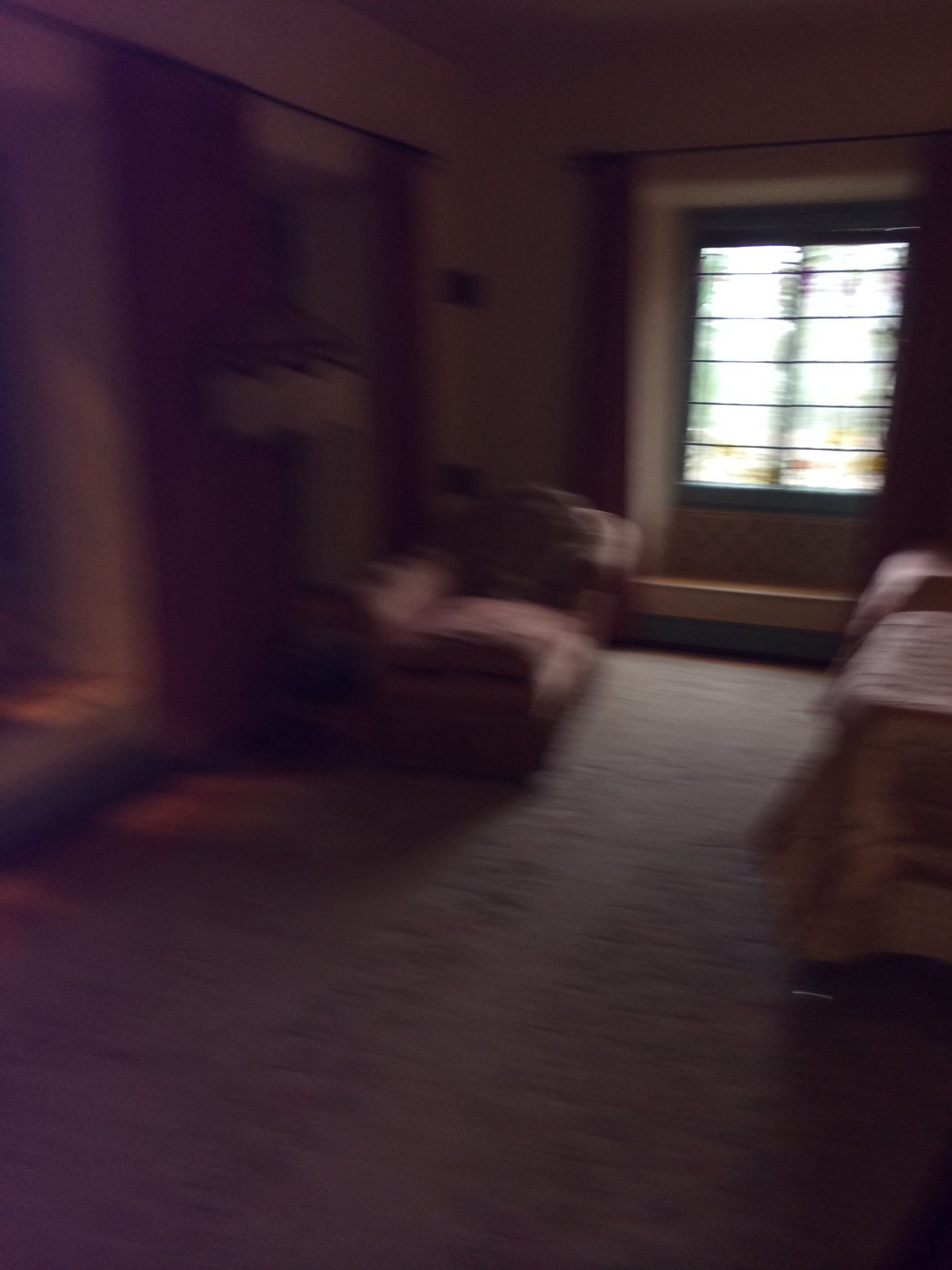The image captures a dimly-lit interior of a home, dominated by darkness and graininess, suggesting it was taken in motion. On the far right wall, a window with five vertical bars allows a limited amount of light to seep in, partially lighting the carpeted floor. The view outside the window is indistinguishable due to the image's blurriness. To the left, what seems to be an entryway is partially obstructed by a sofa, behind which hangs a pole with curtains, indicating a possible window, although the low light masks it from view. On the right side of the image, faint outlines suggest the presence of furniture, potentially a table draped with a tablecloth. A lamp positioned near the curtains behind the sofa (or perhaps a bed) further contributes to the sparse illumination. Harsh shadows cast by the minimal light starkly outline the assorted furniture, reinforcing the room's obscure and mysterious atmosphere.